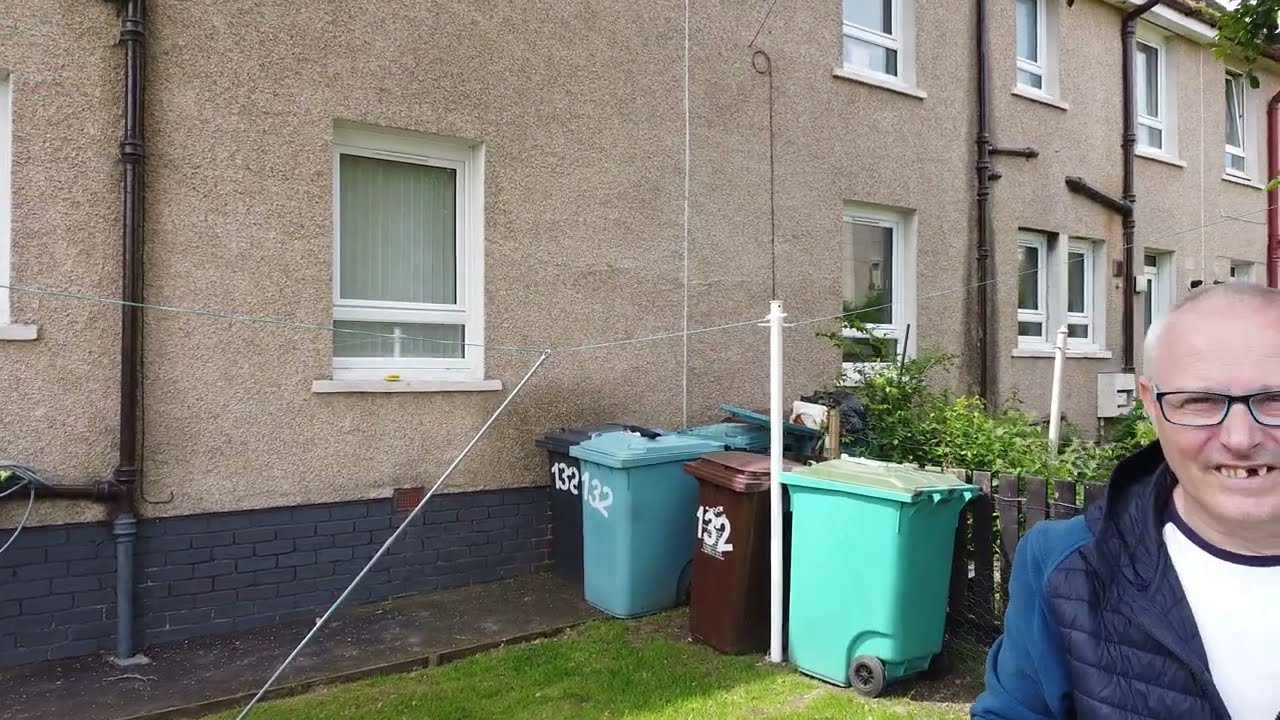In the photograph, a white male with a receding hairline stands on the right, smiling with a noticeable missing front tooth and yellow teeth. He wears thick black glasses, a white shirt with blue trim around the neck, and a blue jacket—dark blue down the chest and lighter on the shoulders. The background features a light brown grimy building with a rough surface. The building has many white-framed windows and a trim of dark blue bricks along the bottom. On the far left side of the building, a brown pipe runs vertically, and in the center, there is a group of plastic garbage cans marked with the number 132. The cans are dark blue, light blue, brown, and teal, with the teal one on black tires and lacking a number. A white pole with wires is also visible between the trash cans. The scene gives an impression of the man having taken a selfie in front of the building, with the garbage cans and a black fence separating the yards adding to the detailed urban setting.